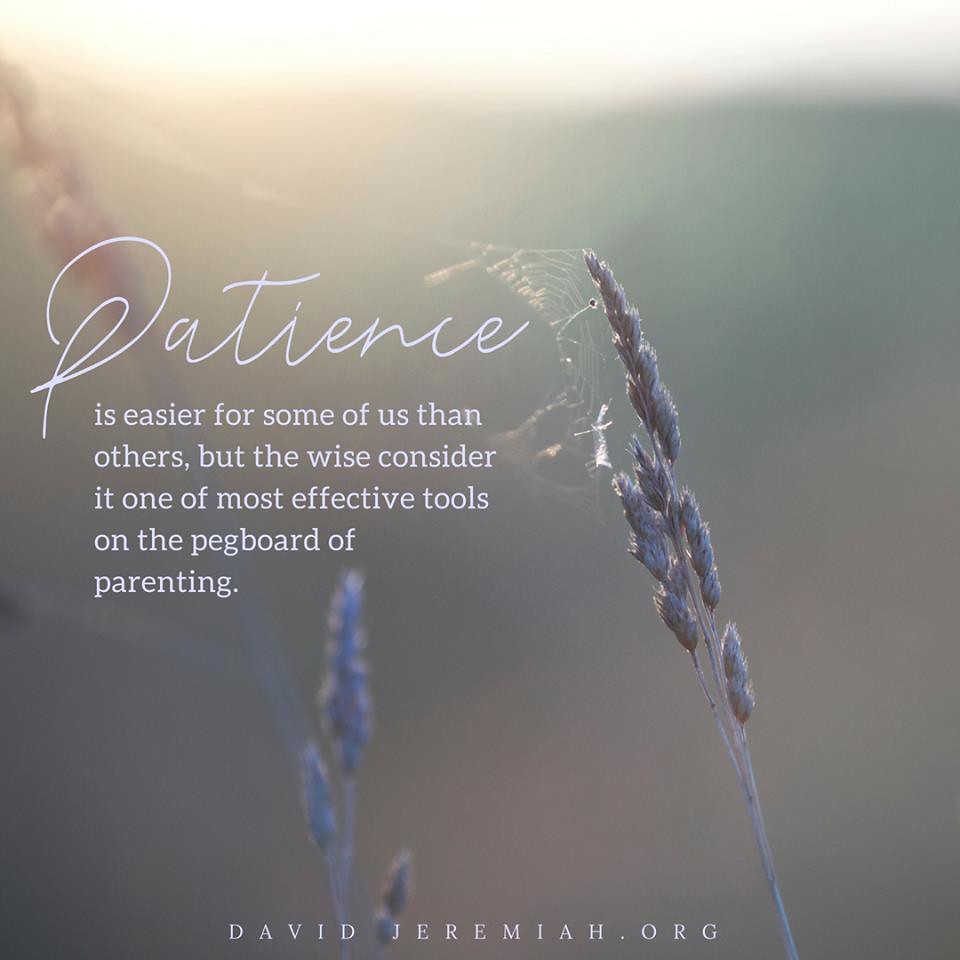The image is a photograph taken at either sunrise or sunset, capturing an ethereal scene where muted shades of gray and light pink blend subtly in an out-of-focus background. The top of the photograph is overexposed, likely capturing the sky, while the middle is dominated by large stalks of grass-like plants. These stalks, which are grayish in color, stretch from the bottom right corner towards the upper left but do not quite reach the center or the top of the frame. A faint, delicately illuminated spiderweb clings to one of the stalks, adding an intricate detail to the composition. 

In the background, the sun casts a warm light, giving the image a serene and captivating ambiance. Over this photograph, there is a quote written in a large cursive font that reads, "Patience." Beneath this, in a white standard font, the text continues: "is easier for some of us than others, but the wise consider it one of the most effective tools on the pegboard of parenting." At the bottom center, a URL reads "davidjeremiah.org," possibly crediting the creator or photographer of the image. This enchanting visual, combined with the thoughtful quote, makes the photograph an inspiring piece that might be fitting for display on a wall.